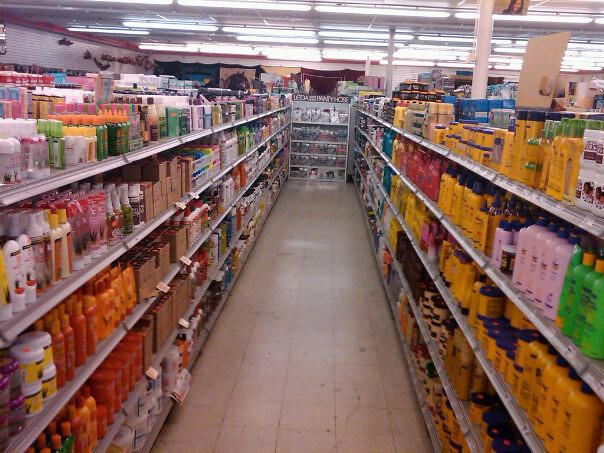This photograph captures the interior of a grocery or convenience store, taken from an elevated perspective at the end of an aisle. The aisle is lined with gray-colored shelving units, adorned with white pricing labels on the front edges of the shelves. These shelves are stocked with an assortment of personal care products, including various types of shampoo, conditioner, and body wash. The items are housed in bottles of diverse colors such as white, yellow, red, pink, orange, and green, creating a vivid display. The store has a tan-colored tile floor and is illuminated by rows of fluorescent tube lights on the ceiling. At the far end of the aisle, a display labeled "LEDA Pantyhose" is visible, also using gray shelving for support.